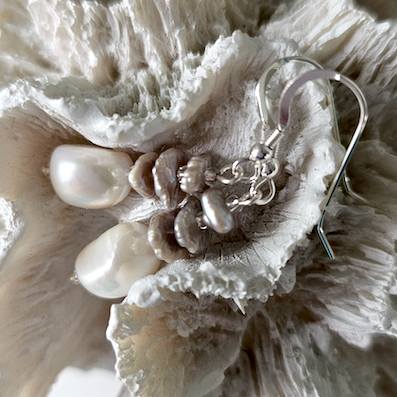The image depicts an elegant set of earrings carefully placed on a soft, white wool-like fabric, giving the appearance of a fluffy, textured rug. The earrings feature a hook at the top that connects to a short chain. Attached to the chain are two slightly flattened, silver round pieces, beneath which dangle two glossy, oval-shaped beads resembling pearls. These pearls are connected to the chain by three smaller round links. The background's wooly texture and the bright natural light enhance the clarity and brightness of the image, making the intricate details of the jewelry and the soft fabric stand out vividly.